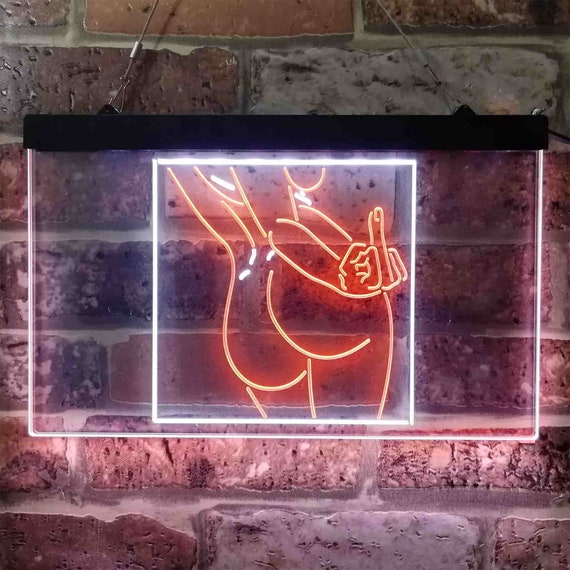The image captures a rectangular, glass-like sign hanging on a standard red brick wall with some white and dark red imperfections. The sign features a black metal or plastic bar at the top, fastened to wires likely anchored by a nail. Inside the glass rectangle, there is a smaller, glowing rectangle made of LED lights designed to mimic neon. This inner rectangle showcases a simple line art drawing of a female form's nude backside, highlighted in red and orange lights, with the cheeks and side of one breast visible. One arm is extended towards the viewer, flipping the middle finger. The image is cropped, cutting off the figure below the middle of the legs and above the shoulders.